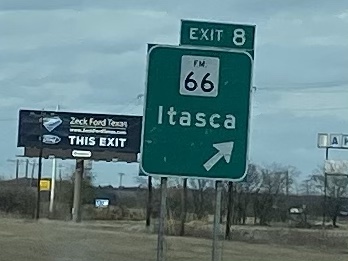The image depicts a highway intersection under a vast blue sky with bluish-gray clouds. The primary focus is on a large green road sign with white lettering. At the top of the sign, situated inside a white box with rounded edges, are the black letters "FM 66." Below this, the sign reads "Exit 8" in large white letters, followed by "Itasca," with a white arrow pointing diagonally to the upper right. Supporting this sign is a gray-brown pole. In the distance, on the left side of the image, a black billboard advertises "Zeck Ford, Texas" with the message "This Exit," accompanied by a diamond-shaped Ford symbol. The landscape appears dry with thin, leafless branches scattered across the scene, and the overall setting is during the daytime.